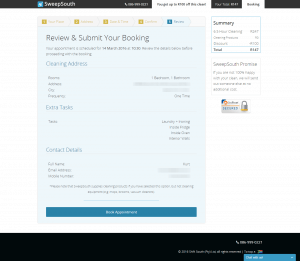This image features a web page from SweepSouth. At the top of the page is a slender black ribbon, displaying the SweepSouth logo on the left in white text beside a bright blue box containing an unreadable icon. To the far right of the ribbon, a white phone icon is shown alongside a phone number. The primary background of the page is a light turquoise blue. Just below the ribbon, there is a row of gray tabs against the blue background, though their labels are unreadable. The text "Review and Submit Your Booking" stands out in large black font, followed by smaller light gray text. Below this, in bright blue text, it says "Clearing Address," with additional gray text underneath. Another section labeled "Extra Tasks" is also presented in bright blue, accompanied by smaller, unreadable information. Near the page's bottom, the section "Contact Details" is labeled, followed by more text. At the very bottom, a bright blue banner spans across the page, containing white text.